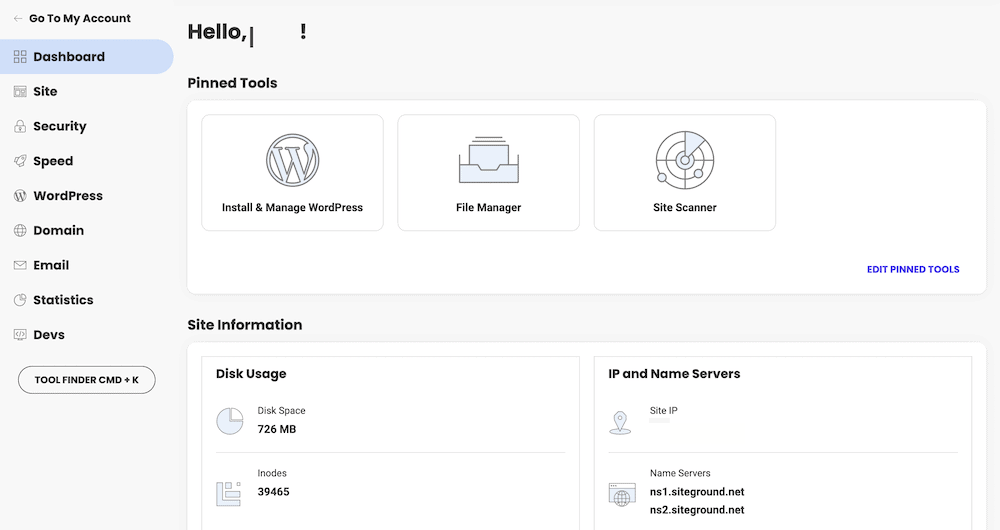In the photographic image, we observe a web page or application interface. At the top of the page, there is a black text instruction reading "Go to my account," accompanied by an arrow pointing to the left. 

On the left side, there is a vertical navigation column. The word "Dashboard" is displayed in bold black font and is highlighted with a blue background. Below it, various menu items are listed: "Site," "Security," "Speed," "WordPress," "Domain," "Email," "Statistics," and "Devs." 

There is a circular button labeled "Tool Finder" with the shortcut "CMD + K." 

To the right side of the interface, a greeting text, "Hello [Name]!" appears, where "[Name]" is left blank and followed by an exclamation point.

Pinned tools are displayed in three distinct boxes. The first box is titled "Install and Manage WordPress," marked with a circular "W" icon. The second box, labeled "File Manager," shows a file box with blue file icons. The third box, "Site Scanner," features a radar-like circular icon. Under these pinned tools, there is a blue hyperlink labeled "Edit Pinned Tools."